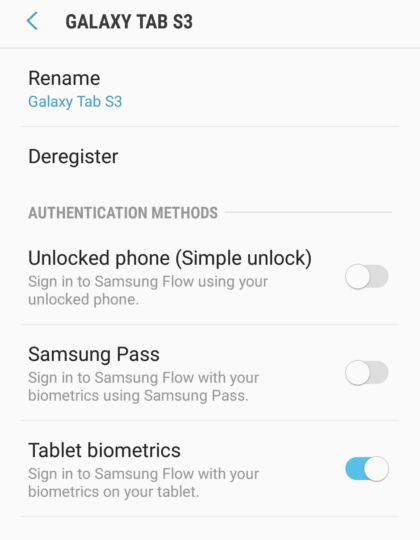Screenshot of Samsung Galaxy Tab S3 Settings Page:

At the top of the screen, "Galaxy Tab S3" is prominently displayed. To the left of this text, there is a blue back button. Below this header, a line divider separates the sections.

The first section features the option to rename the device. "Rename" is in black text, and below it in blue text, it states the current name: "Galaxy Tab S3."

The next section is "Deregister and Authentication Methods."

Following that, the "Unlock Phone (Simple Unlock)" section includes smaller gray text that explains: "Sign in to Samsung Flow using your unlocked phone." To the right of this text is a gray toggle button, which is currently in the "off" position.

Below this is the "Samsung Pass" section, which states: "Sign in to Samsung Flow with your biometrics using Samsung Pass." The toggle button here is also gray and in the "off" position.

The next section is "Tablet Biometrics," which allows signing in to Samsung Flow with tablet biometrics. The toggle button in this section is blue and in the "on" position.

The entire page features a light gray background, maintaining a clean and minimalist design.